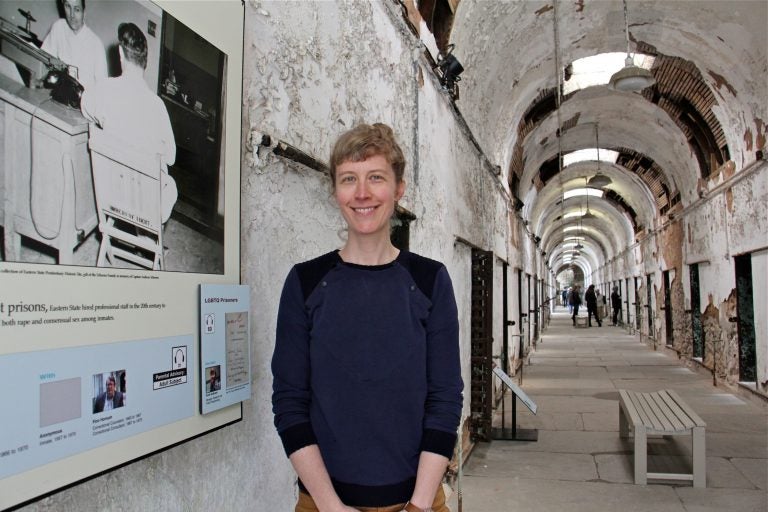The photograph captures a young woman with a short pixie haircut, wearing dark blue sweater and brown pants, posing and smiling for the camera. Her sleeves are pulled back to her elbows, revealing a light brown wristwatch, and she stands with her arms crossed at her waist, showcasing a friendly demeanor with her upper row of white teeth visible. In the background, the scene is set in what appears to be a historical museum housed in a dilapidated, war-torn building with a domed ceiling and a wide hallway. The walls, which were once painted white, now have much of the paint and plaster fallen off, exposing white and tan-colored bricks. There are multiple doorways with grated bars, possibly indicating prison cells, as suggested by the prominent word "prisons" on a poster beside the woman. This poster also features an image of a man at a desk with another man facing him, hinting at interrogation or polygraph scenarios. Scattered along the hallway are several pictures and plaques, and a plain slat bench is positioned to the right. The hallway also contains a short gray bench in its center, and a few visitors can be seen in the far background, adding to the museum-like ambiance of the setting.